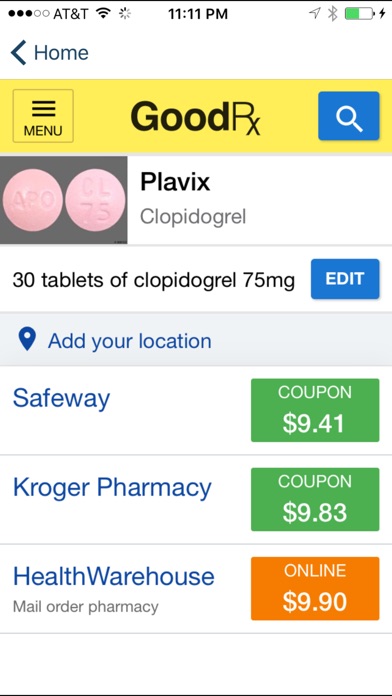The image depicts a smartphone screen displaying the GoodRx website late at night at 11:11 p.m., with the phone operating on the AT&T network. The battery icon on the right side of the status bar indicates that the battery is at roughly 50% capacity, highlighted in green, alongside full internet connection bars.

The header of the GoodRx website includes a yellow navigation bar with "Home" accompanied by a left-pointing arrow on the far left, and the GoodRx logo prominently centered in black text. In the same header, a blue square containing a search icon is positioned on the right, and a yellow square labeled "Menu" is on the left.

Below the header, two pink pills are shown beside the text "Plavix," which is followed by the generic name "Clopidogrel." The listing specifies that it is for 30 tablets of Clopidogrel at a dosage of 75 milligrams. To the right, there is an "Edit" button inside a blue box with white text.

Further down, a prompt to "Add your location" is displayed alongside a pin icon. Subsequently, there are price listings for the medication at various pharmacies: Safeway offers a coupon for $9.41, Kroger Pharmacy for $9.83, and Health Warehouse (an online mail-order pharmacy) for $9.90. The prices for Safeway and Kroger Pharmacy are shown in green boxes, while the Health Warehouse price is highlighted in an orange box.